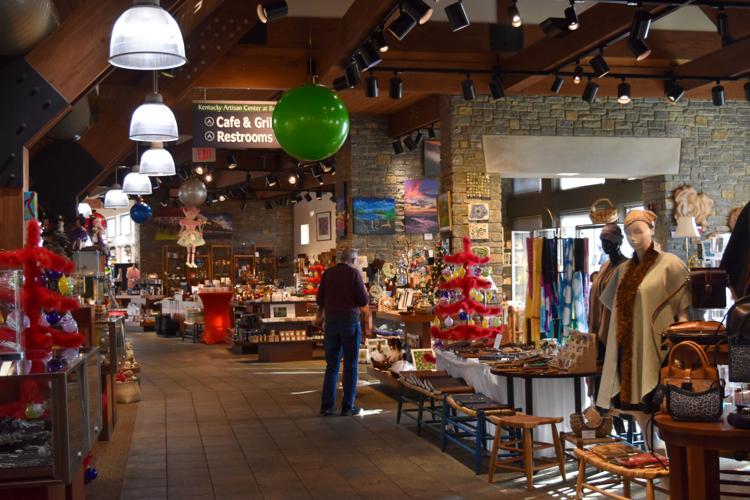The image captures the lively interior of a Kentucky Artisan Center, resembling a bustling indoor market or rest stop. The space is characterized by a cobblestone or brick-paved walkway flanked by a myriad of small shops on either side, each bursting with colorful goods ranging from accessories to vibrant Christmas-themed items. There's a prominent sign that reads "Cafe and Grill" and points to the restrooms, suggesting this is a popular tourist destination.

Overhead, exposed wooden beams and black spotlights highlight various parts of the market without overwhelming the atmosphere. The walls are adorned with a mix of stone facades and plain white segments, contributing to a rustic, yet inviting ambiance. White lights hang down, further illuminating the diverse array of merchandise.

A notable element is an older gentleman with graying hair, dressed in blue jeans, black shoes, and a maroon or red long-sleeve shirt. He stands alone in the midst of this vibrant setting, seemingly engrossed in exploring the items for sale. A mannequin dressed in a tan cape and hat, glass display cases filled with various goods, and shelves stocked with food items add to the eclectic and colorful scene. This image captures the essence of a busy market, albeit momentarily quiet, with just one shopper.